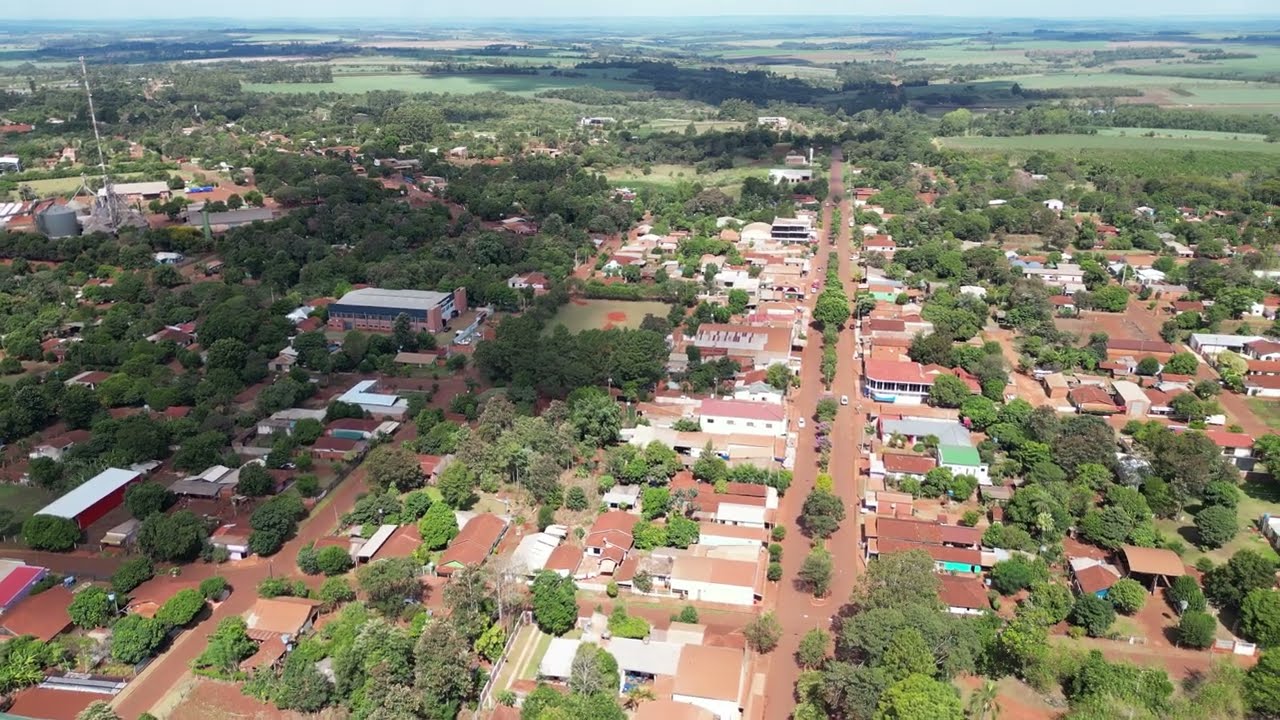An aerial photograph, most likely captured by a drone, showcases a picturesque residential area of a town. The view encompasses a street extending into the distance, flanked by numerous single-story houses, each featuring distinctive orange-tiled roofs and white exteriors. The street, with its brown or reddish-brick surface, is lined with trees both along its lanes and intermixed among the homes, creating a lush and verdant atmosphere. Toward the left corner of the image, a tall antenna—possibly associated with a radio station—stands out, accompanied by a red barn or warehouse. As the street stretches further, the dense urban sprawl gradually transitions into expansive grassy valley areas, bordered by gentle hills in the background. The photograph, taken during the daytime with the sun shining through a partly cloudy sky, captures the rich greenery and orderly layout of this serene and vibrant neighborhood.